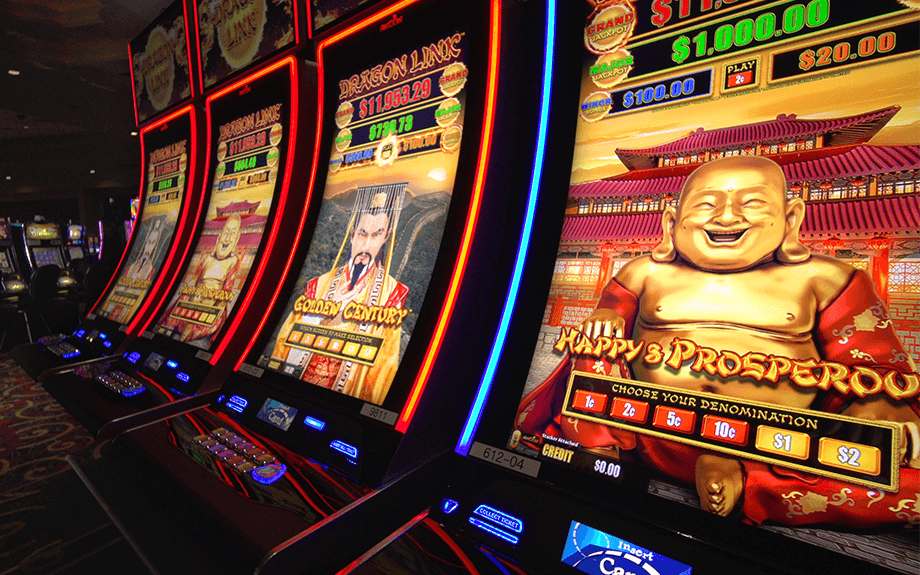This image captures a row of illuminated slot machines in a dimly lit casino environment. The focal point is four slot machines arranged side by side, with a few more visible in the background. The machines are adorned with vibrant colors, bright LED lights, and neon accents that enhance their visual appeal. The first machine features a gold-colored Buddha with a smiling face, elongated ears that touch his shoulders, and a chest radiating white light. This Buddha is set against the backdrop of an Asian-style house with the text "Happy Prospero" and "Choose Your Denomination" displayed. The denomination options include red buttons for 1¢, 2¢, 5¢, and 10¢, along with yellow buttons for larger bets like $1 and $2. Above these buttons are rectangles indicating prize amounts: $1,000 in black, $100 in blue, and $20 in orange. The next machine introduces a fierce-looking samurai, holding swords, with a black goatee and a thin mustache, under the label "Golden Century." This pattern of alternating imagery continues down the line, with another golden Buddha and another samurai-themed machine, contributing to the vibrant and thematic array of gambling entertainment.